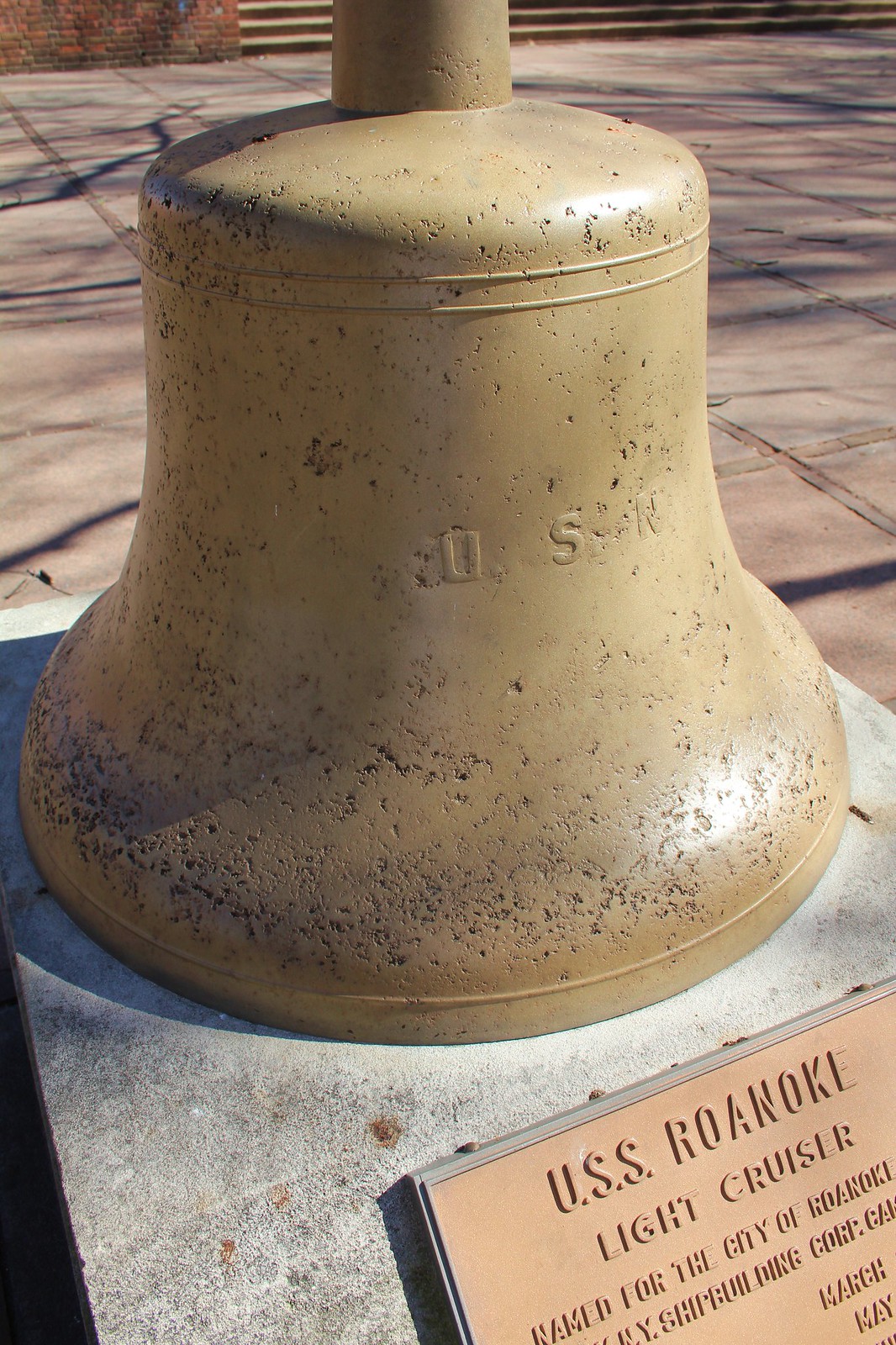The tall, rectangular photograph features a statue resembling an upside-down bell, which is predominantly beige in color. The top of the statue is cut off and a pole-like protrusion extends beyond the image. This bell-like structure sits on a smooth, gray cement or stone base, which is cropped on the left and bottom edges of the photo. In the bottom right corner of the base is a partially visible copper-colored plaque with a silver border. The legible part of the plaque reads "USS Roanoke Light Cruiser." The background reveals a reddish-brown tiled walkway and a distant red brick wall with a set of stairs.